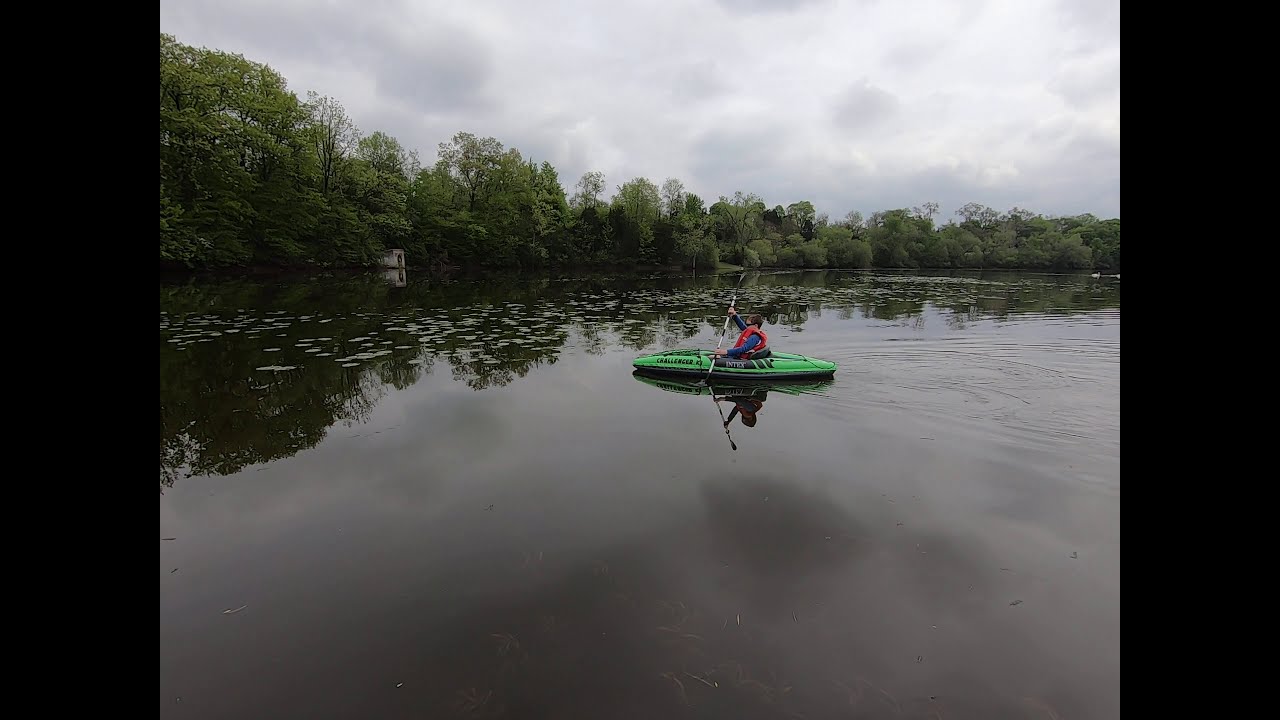In the very center of the image, a boy with brown hair and sunglasses is actively paddling a bright green and black kayak labeled "Challenger" in black letters, with "Intex" in white further along the side. He is wearing a blue long-sleeve shirt and a red life vest as he navigates through a patch of lily pads on a dark, still body of water. His left paddle is immersed in the water, indicating he is in motion. Surrounding him on the left and curving around to the rear are lush, green bushy trees. To the right side of the waterbed, a white-colored boathouse or shed emerges amid the dense treeline, barely visible. The sky overhead is a soft, stormy gray, enhancing the tranquility of the scene. There is foamy residue on the left side of the water, suggesting a boat recently passed through. The image is framed by some black rectangles on the left and right sides, focusing attention on the boy in the kayak.